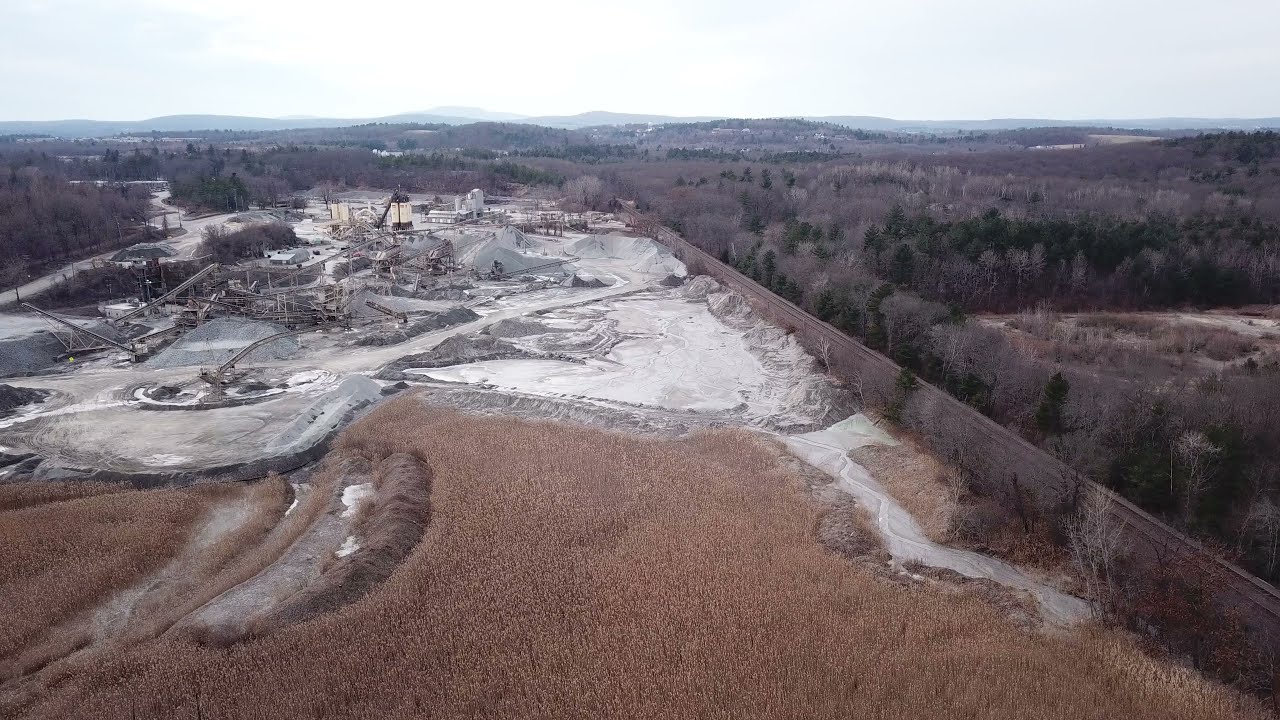This aerial photograph captures a detailed view of a landscape featuring a blend of nature and industrial activity. Central to the image are railroad tracks cutting through the scene. To the right of the tracks lies a densely wooded area, rich with trees in various stages of foliage—some vibrant green and others barren, indicating the late autumn or early winter season.

On the left side of the tracks, a construction site is evident. The site appears to be involved in mining or excavation activities, with piles of light-colored dirt or gravel scattered around. Construction buildings and equipment are visible in the background. A white sand or rock area suggests extensive digging operations. The presence of a wall or fence running along the right side adds to the logistical layout of the area.

In the distance, the terrain transitions into a golden-colored wheat field, creating a stark contrast with the industrial site. Distant mountains form a backdrop with a cloudy sky overhead, hinting at an overcast day with limited sunshine. The photograph captures the juxtaposition of natural beauty and human industry, framed against a moody sky.